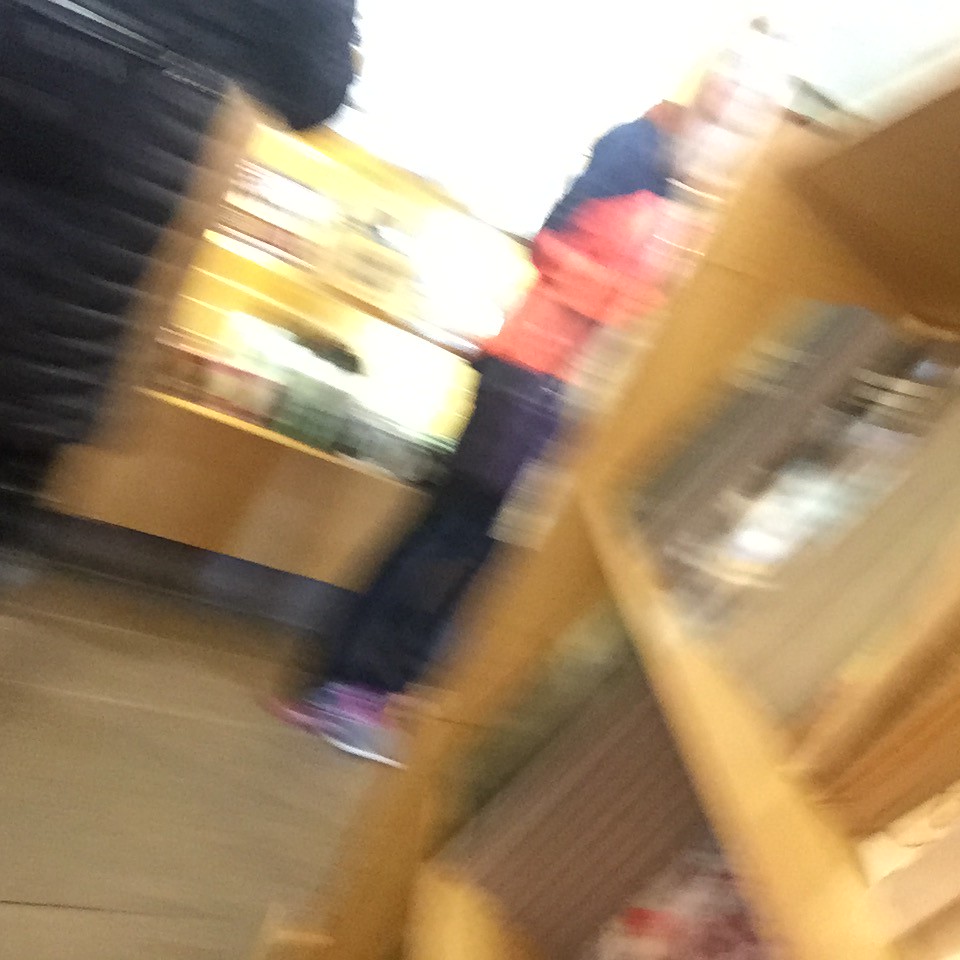This color photograph appears to have been taken indoors and is significantly out of focus, making details difficult to discern. It seems to depict a scene in a well-lit space, possibly a bookstore, with sunlight streaming in through a window with partially open blinds. A bookcase stands prominently on the right side of the image, filled with books on the top and second shelves. Among the blurred figures, one individual stands behind the bookcase, dressed in a black and red long sleeve shirt, dark denim blue jeans, and grey shoes. Another person is positioned next to the window, possibly wearing a black shirt. In the background, there are hints of additional shelving or counters made of light tan wood, and the flooring appears to be made of large light brown tiles or stone. Despite the clarity issues, the scene is brightly lit, with some areas of the photograph overexposed to white.